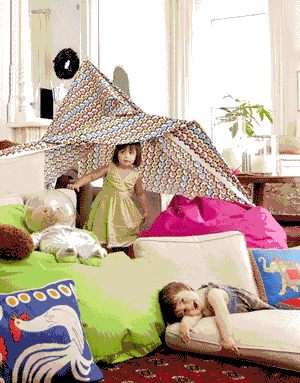In this warmly-lit photograph, two toddlers are engrossed in play within their homemade indoor fort, set against the backdrop of white walls. On the left, a tall mirror reflects part of the scene, while a large window with white curtains on the right lets in soft, natural light. At the center of this cozy adventure space is a vibrant, tent-like canopy made from colorful bed sheets, forming a whimsical play tent. Peeking out from beneath the fabric canopy is a little girl in a green dress, standing between a pink beanbag and another green beanbag. Nearby, a boy, facing the camera, is comfortably sprawled on white cushions, adding to the scene's playful ambiance. A stuffed animal rests atop one of the beanbags, completing this charming, campsite-like setting within their home.